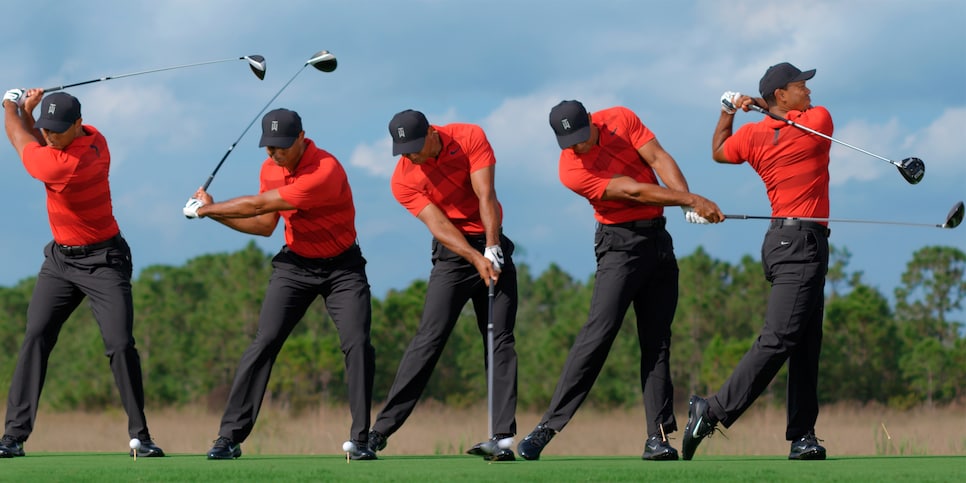The image captures a series of five sequential shots of a golfer, who closely resembles Tiger Woods, executing a golf swing on a bright, clear day. The background features a vivid blue sky with hints of white clouds and a verdant line of large green trees. In the foreground, the well-manicured, smooth green of the golf course is visible along with patches of light tan tall grass.

The golfer, dressed in a bright red-orange shirt, black hat with the initials "TW" in white, black pants, black shoes, and a white glove on one hand, is shown in five distinct phases of his golf swing. From left to right, the first image displays him pulling his golf club back. The second image captures the club at its peak height. In the third image, the club is at the bottom, moments before striking the ball. The fourth shot shows the golfer mid-swing. The final image captures the golfer in his follow-through posture, with the club swung back around. The bright and clear setting enhances the overall clarity of the image, emphasizing the fluid motion of the golfer’s swing.